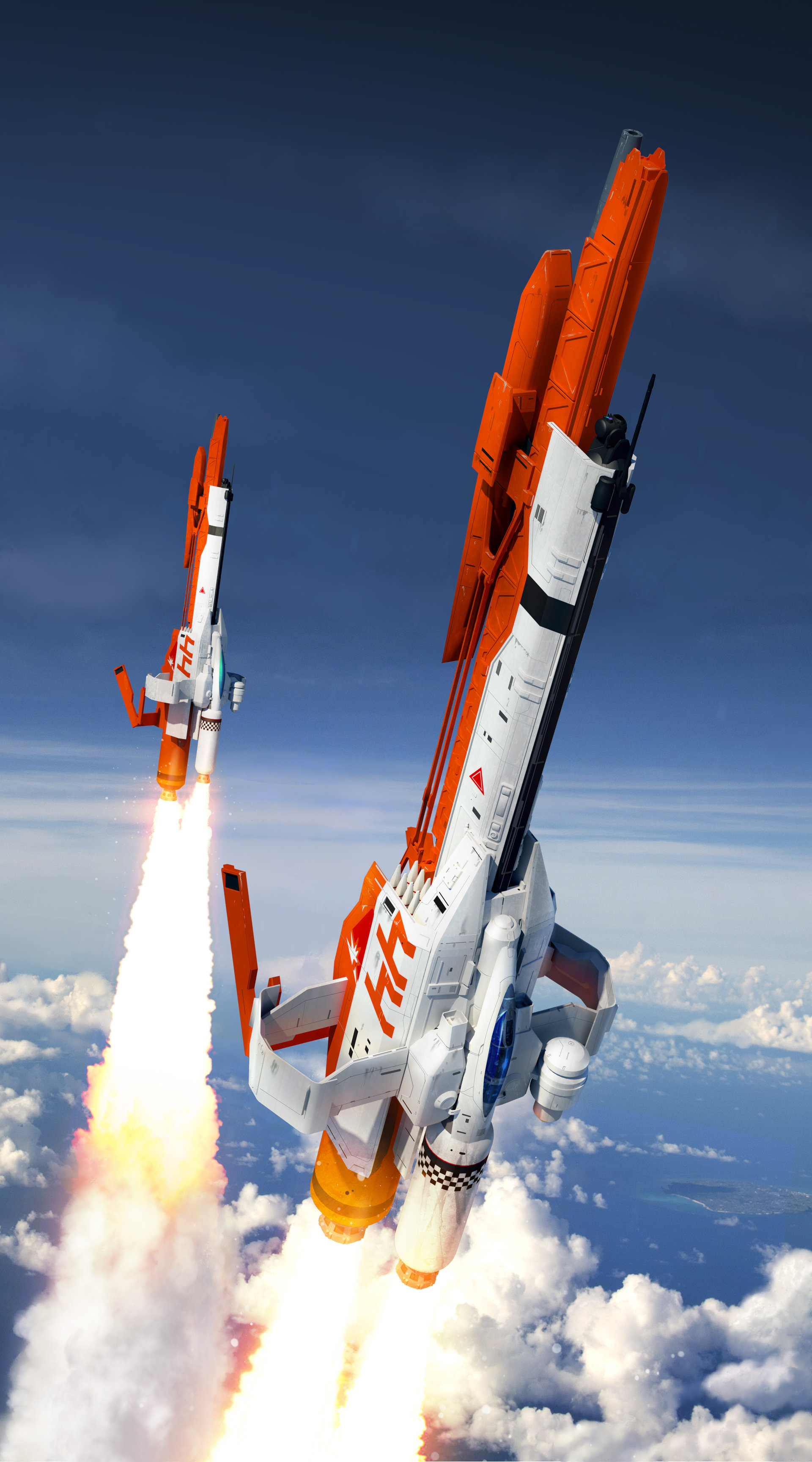In this upright, rectangular image, two rockets are captured mid-flight as they launch into space, ascending through a gradient sky that transitions from dark blue at the top to lighter blue lower down, with a layer of fluffy white clouds beneath them. The rockets are seen above the cloud cover, yet still within the Earth's stratosphere or atmosphere. Each rocket has a distinctive design, primarily white-bodied with red tips and trim, accentuated by bright orange blasters emitting plumes of fire and smoke. The rockets feature prominent red "H" markings on their sides alongside a large red triangle pointing upwards. The rocket positioned in the foreground appears larger, though this could be an effect of perspective, with the second rocket slightly smaller and to the left. Both rockets resemble futuristic spacecraft, evoking imagery akin to Star Wars ships or even large guns due to their unique shape and design.